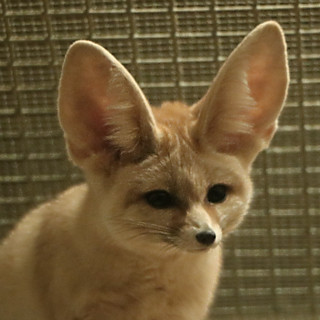In the image, there is a fennec fox positioned centrally against a backdrop that appears to be a metallic cage characterized by a grid pattern of horizontal and vertical wires. The fox's fur is predominantly a light sandy beige color with slight variations of darker beige, giving it a golden hue in some areas. Notably, the fox has enormous, erect ears that are almost as large as its body, with some fur visible along the inner edges. Its features include very dark, beady eyes, a tiny black nose, and black whiskers adorning its thin snout. The area between its ears shows a slightly darker shade of fur, adding to the detail of its coat. Overall, the image captures the distinctive and striking appearance of the fennec fox within its enclosed habitat.